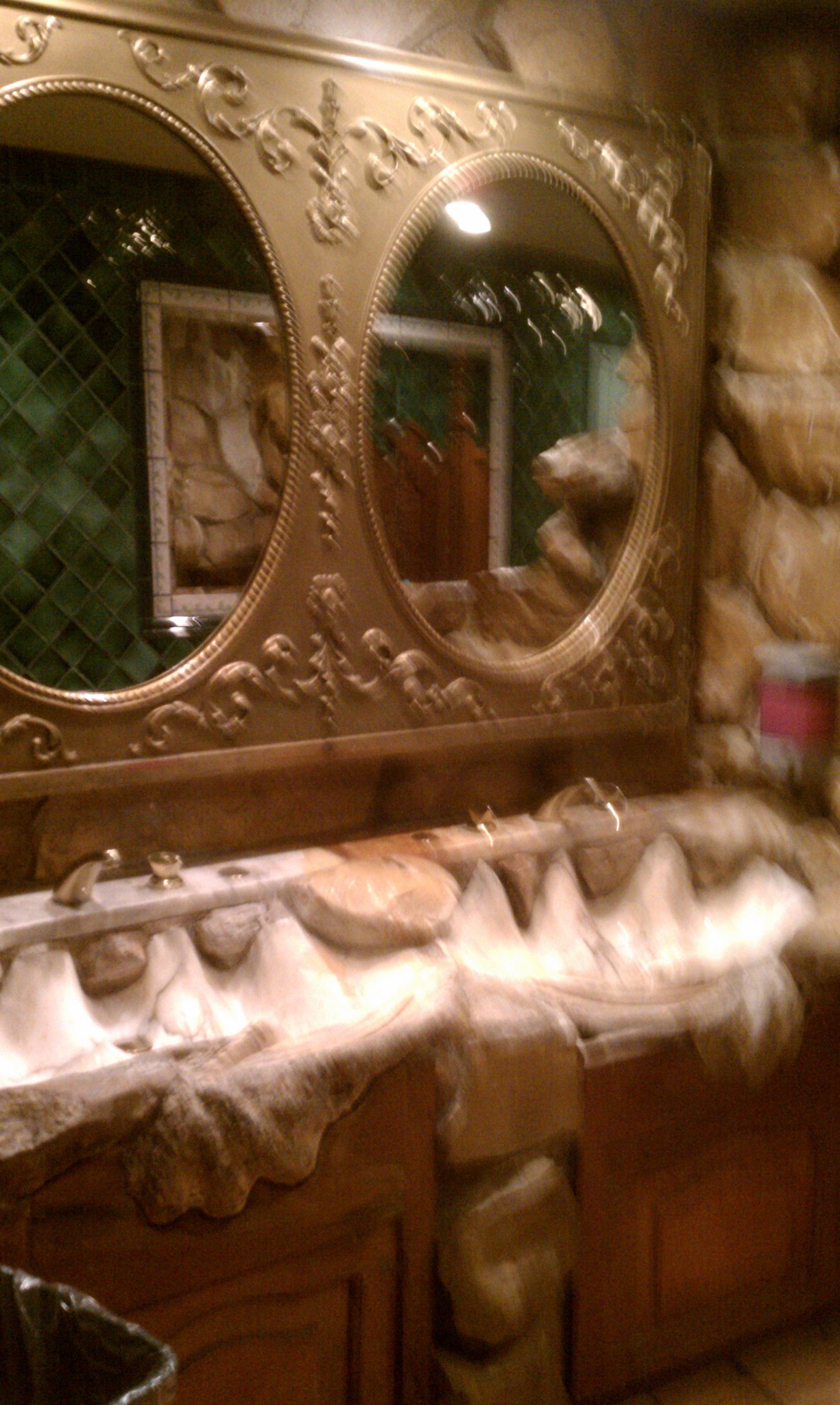The image depicts the slightly out-of-focus interior of an upscale bathroom, possibly in a high-end restaurant or commercial building. The focal point is a unique sink area crafted from wavy stone or river rock, designed to resemble giant seashells, sitting atop a wooden cabinet with drawers. The walls are adorned with large, tan cobblestone-like river rocks, enhancing the natural, rustic aesthetic. Above the sink, two ornate, oversized oval mirrors framed in gold or bronze with intricate, swirling designs hang on the wall, adding a touch of elegance and opulence to the space. In the reflection of the mirrors, there are indistinct views of a door, some tiles, and possibly a picture on the wall, further indicating the bathroom setting.